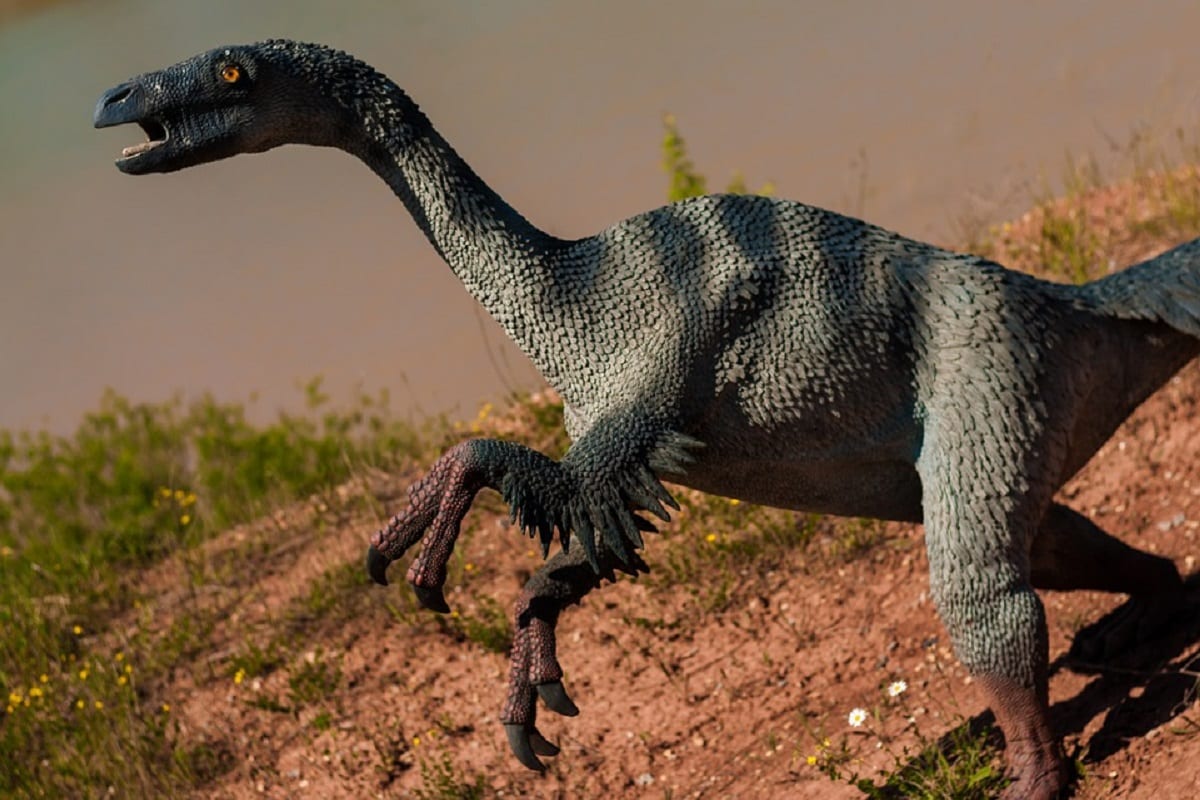The image depicts a detailed, lifelike statue of a green dinosaur, possibly a raptor, positioned in a natural outdoor setting. The dinosaur, which appears to be scaly with a few feather-like structures, has a long neck and walks upright on two back legs, while three large claws protrude from its front limbs. The creature's eyes are striking, one being described as orange and another as golden, with an open mouth revealing a pink tongue. The dinosaur stands on a dirt-covered hill adorned with small yellow flowers and green weeds. The ground shows patches of reddish and brown earth, contributing to the naturalistic setting. In the background, the sky mixes hues of gray to blue, creating a contrast with some visible grass and distant plants, enhancing the realism of this 3D-rendered or sculpted prehistoric scene.